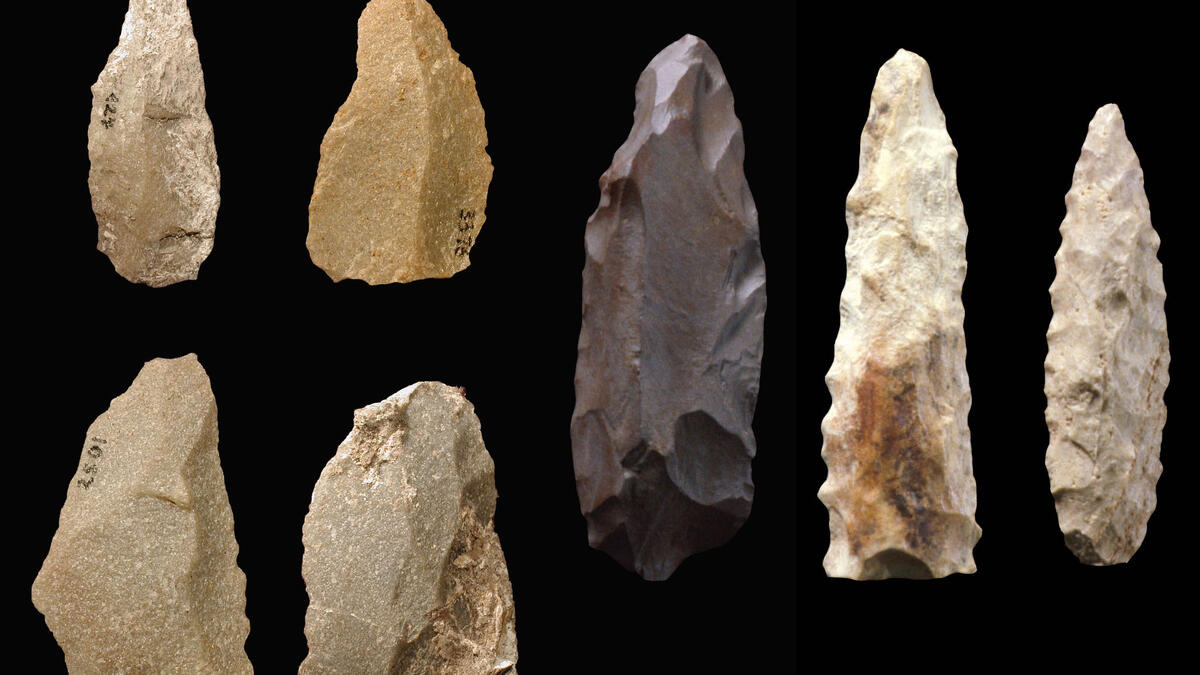The image displays seven distinct objects against a stark black background. These objects resemble arrowheads, potentially crafted from flint or similar stone materials. On the far left, there are two smaller, oblong arrowheads positioned towards the top, both a tan color, with the left one slightly lighter. Below them, partially cut off at the bottom, are two more light tan arrowheads of a similar shape. Moving towards the right, there is a very dark, almost black arrowhead centrally placed. To the right of this, there is a white arrowhead with a hint of brown. The far-right side of the image features a smaller, teardrop-shaped arrowhead. Each arrowhead is intricately chipped around the edges, underscoring their handcrafted nature. The uniform black background serves to highlight these seven varying arrowheads, emphasizing their details and differences in size, shape, and color.